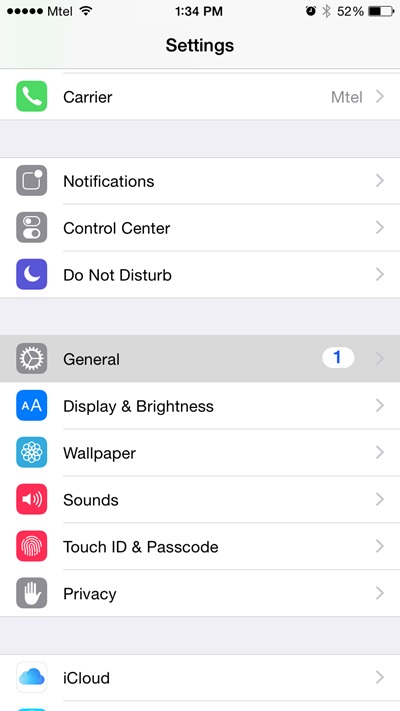The image appears to be a screenshot of an iPhone displaying the Settings app in Portrait mode. In the status bar at the top, there are five black circles followed by "MTEL" indicating the carrier. The Wi-Fi icon shows full signal strength with all three bars filled. The time displayed is 1:34 PM. Other icons include an alarm clock symbol and a grayed-out Bluetooth symbol. The battery indicator shows 52% remaining, displayed horizontally.

Below the status bar, the screen includes the main sections of the iPhone's Settings app with corresponding icons on the left side of each option and right-pointing arrows indicating further menu options. The visible settings options include:

- Notifications
- Control Center
- Do Not Disturb
- General

To the right of the "General" option is a rectangular button with rounded corners labeled "1," likely indicating a notification or update.

Further down, additional settings options displayed are:

- Display & Brightness
- Wallpaper
- Sounds
- Touch ID & Passcode
- Privacy
- iCloud

The next row is partially visible with just a portion of the corresponding icons and text. Each row features an icon to the left and most rows have right-pointing arrows indicating submenus or further settings information.